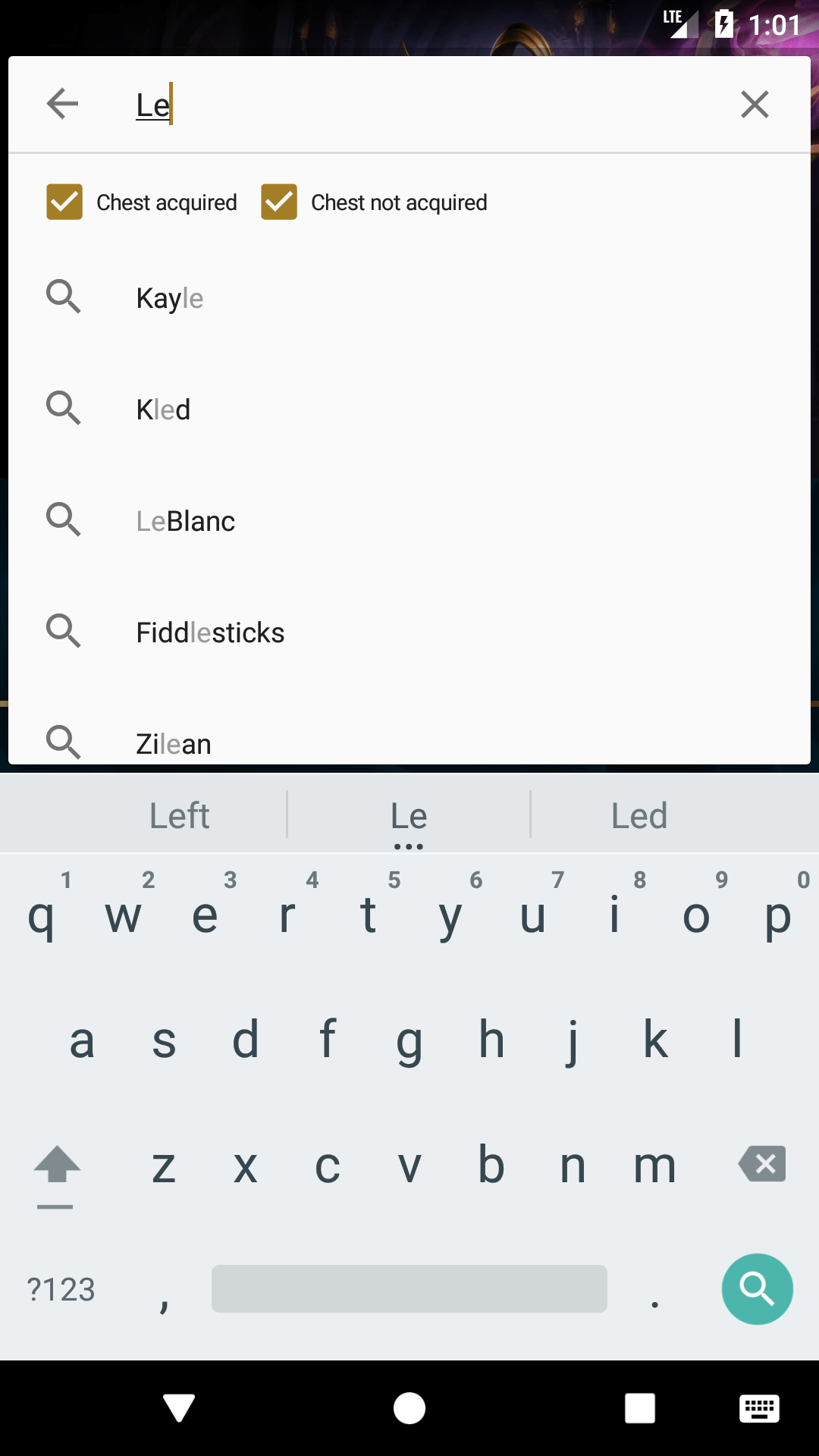A detailed product features listing image is shown with various electrical and hardware components. It includes a USB-C port labeled clearly, indicating Electro technology compatibility and LTE connectivity. The battery status is displayed at 101%, alongside a checkmark signifying that trust has been acquired for the device or software. Additional items and features include icons and text references to "Trust Not Acquired," accompanied by a magnifying glass labeled "Manifind Glass" and "Kailh," indicating a detailed inspection feature for switches or keys.

Highlighted components consist of display types like "Manifind Glass KLED," "Natural Glass LeBlanc," "Manifind Glass Fiddle Sticks," and "Manifind Glass Alien," possibly denoting specific glass or display technologies. There are instructions or meaningful areas pointed out as "Where This Is Left" and "Where It Says LED," accompanied by sequences of characters like "123456790," "QWERTYUIOP," and "ASDFGHJKL," likely referring to keyboard layouts or test input sequences.

Additional labels include "Shipped Up," identifying possibly shipped status or package orientation, and "Says DXDBBNM," which could be part of a diagnostic test or setup process. A backspace function highlighted with "Backspace With Exit," followed by a "Question Mark," sets focus on navigational or help features. Shapes such as a gray rectangle, a blue circle, another "Question Mark," a magnifying glass marked "Manifind Glass," a black bar, a white down arrow, a white circle, and a white square are also present for further symbolic instruction or indication.

Overall, the image meticulously labels and describes various aspects and functionalities of a highly technical and detailed product or device interface.